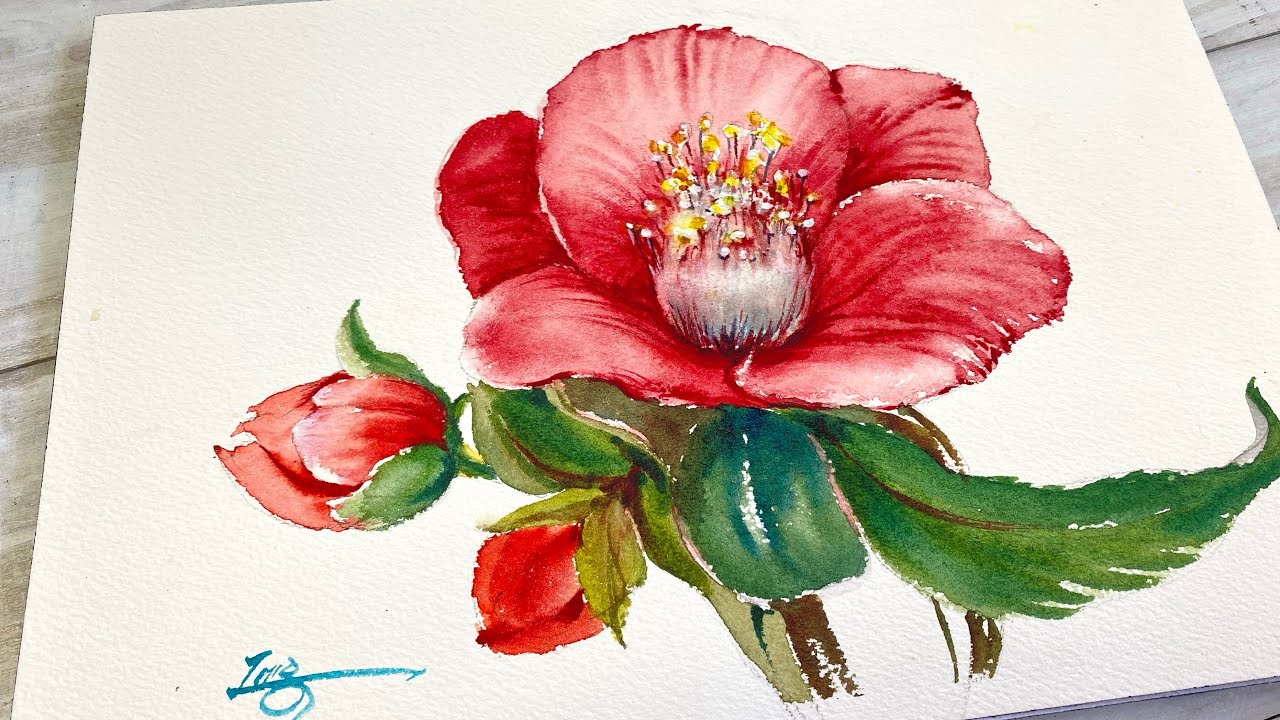This detailed watercolor painting depicts a vibrant red rose with five petals, prominently displayed in the center of a roughly textured, off-white paper. The rose features three main red petals with pink highlights on the edges that converge in the middle, subtly overlapping with two others partially concealed underneath, creating a layered effect. The center of the rose is adorned with yellow-tipped stamens reaching upward from a fuzzy white ball. Surrounding the main rose are deep green leaves, some with a slight yellowing and brown tint near the buds on the lower right. Additionally, there are two unopened buds, one extending directly to the left and the other positioned diagonally beneath it. The bottom left corner of the painting bears a stylized signature in blue, starting with a 'T' and ending with a 'G,' though the exact name remains uncertain. This piece lies atop a light brown wooden surface, possibly a table, adding to its natural presentation.